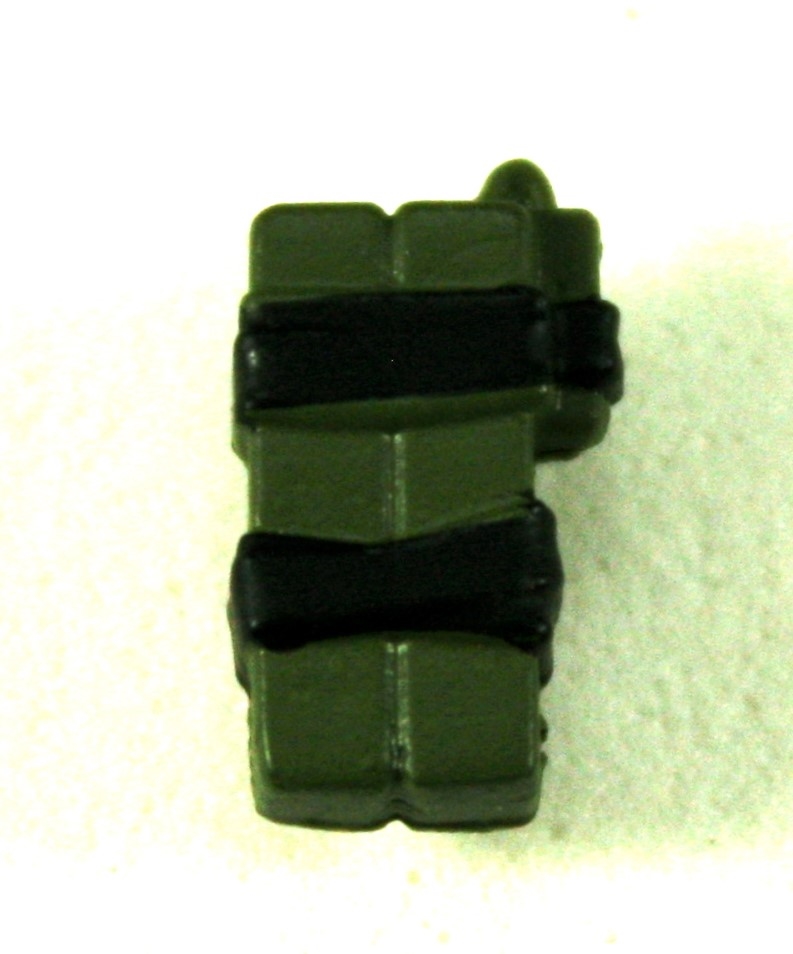The photograph depicts a mysterious green object composed of multiple rectangular shapes, which appear to be either plastic or metal. The main body of the object consists of two long, bright green vertical rectangles that are intersected by two dark green horizontal bands, seemingly holding the structure together. Additionally, a darker green rectangular piece extends vertically from the right side, connected to the other parts. The overall construction suggests that it might be an assembled object, reminiscent of the green foam used for floral arrangements but more rigid and compact. The background is indistinct and blurry, featuring a predominantly washed-out white surface with a rough texture and faint detailing, possibly speckles or tiny holes, most noticeable in the lower right corner of the image. The surface appears light green with a rugged feel, though it is largely obscured in the photograph.